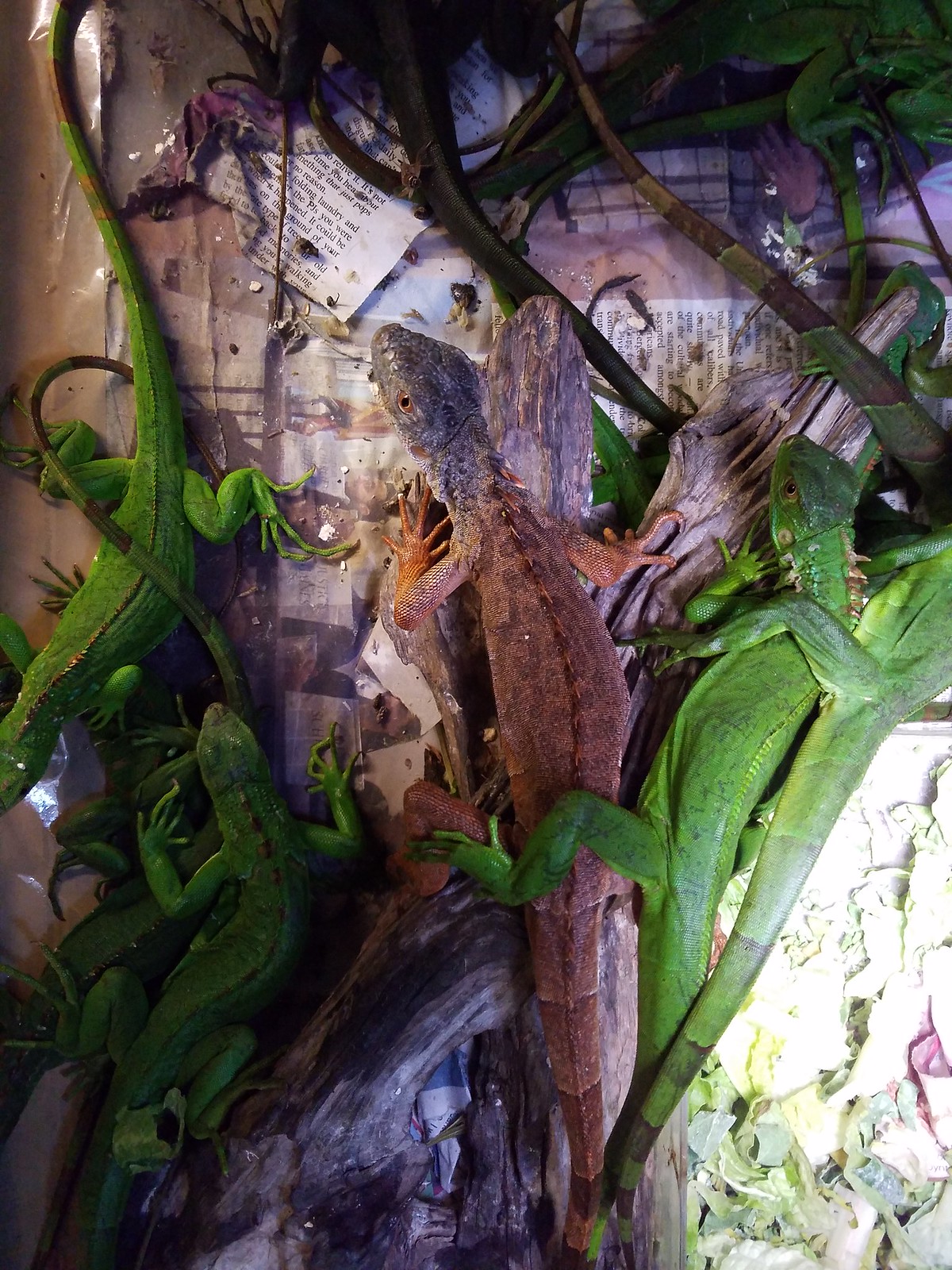This detailed portrait-oriented color photograph captures a group of six iguanas, positioned on top of a surface that includes newspaper and wooden logs, with some plastic baggies, branches, and leaves scattered around. Taken from an overhead perspective in a somewhat dimly lit scene, a bright light shines on the grass to the right of the frame. In the center of the photograph, a long brown iguana is prominent, vertically oriented with its head towards the top. This brown lizard has a green iguana resting on its back, with a leg extended over it. Additionally, another green iguana is precariously perched atop the first green one. On the left side of the brown lizard, two more green iguanas are seen; one is facing downward with its head disappearing off-frame, and beneath it, another lizard faces upward. To the right of the brown iguana are two more bright green iguanas, partially stacked, with the lower body's left leg extended over the other. The iguanas seem to be intertwined, creating an intricate composition that highlights their vibrant green and brown hues amidst the mixed background elements.